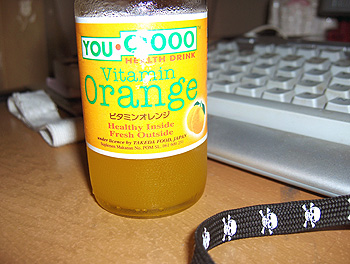Side view of a wooden desk with a brown surface. On the left side of the desk, there's a black lanyard adorned with white skulls and bones. Positioned centrally on the desk is a grayish keyboard; the letters N, V, H, and the spacebar are visible but the rest is slightly blurry. To the right of the keyboard, there is a clear glass bottle containing an orange drink. The bottle features mostly orange packaging with a white strip at the top and bottom. The label includes a partially illegible green logo starting with a 'U', followed by '000' and 'orange health drink'. Additionally, it mentions 'vitamin orange' and some Asian characters that are not readable.